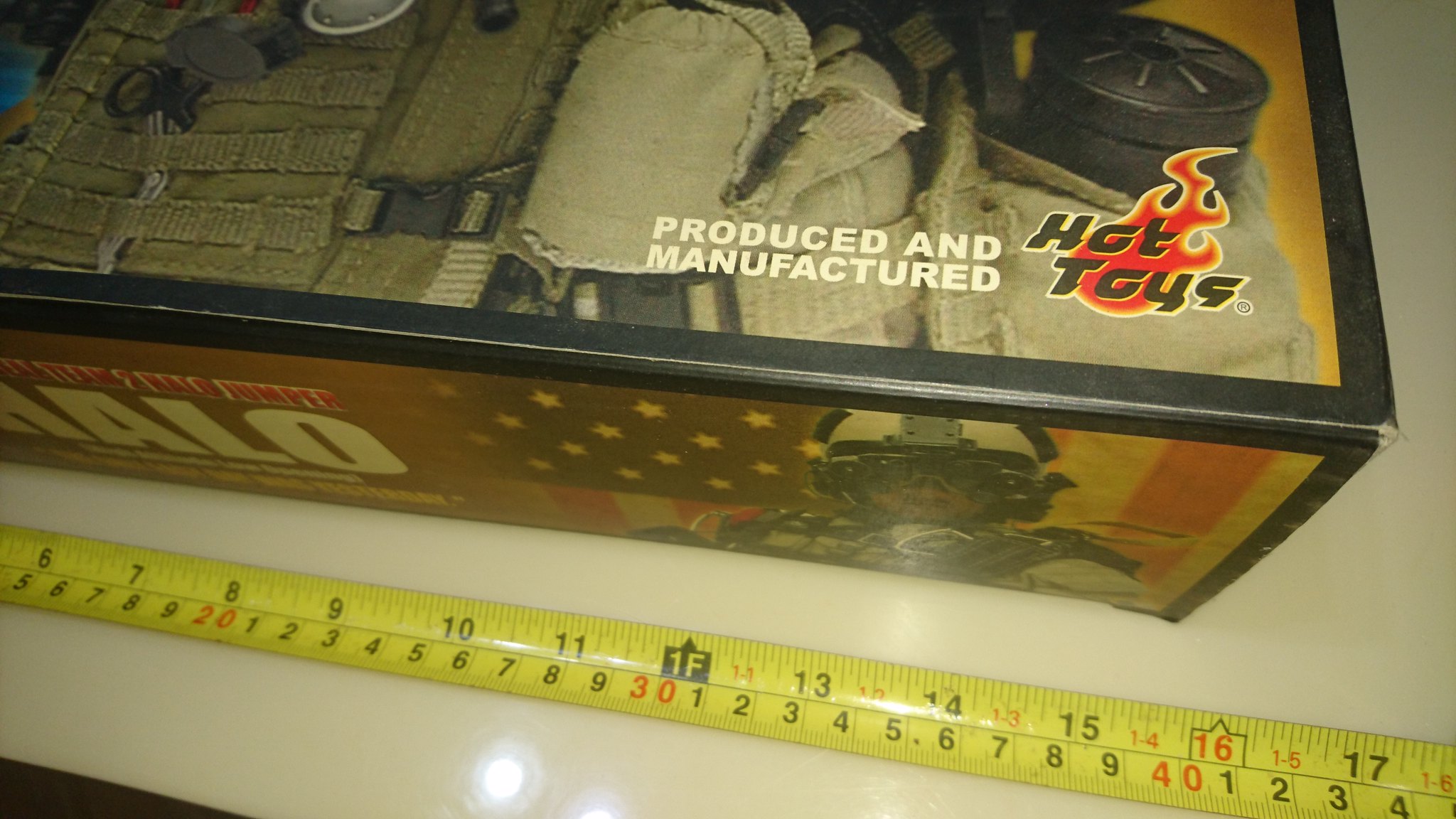On a white tabletop speckled with small brown spots, a bright yellow measuring tape with black and red numbers is laid out. Atop the table sits a prominently placed box. The box is primarily brown with a distinct black outline. On its surface, white letters spell out "Produced and Manufactured" alongside a red flame icon bordered in yellow that reads "Hot Toys" in bold black font. The side of the box features the word "Halo" in white letters. In the background, part of a flag is visible along with an individual wearing a white and gray helmet, reminiscent of motorcycle gear.